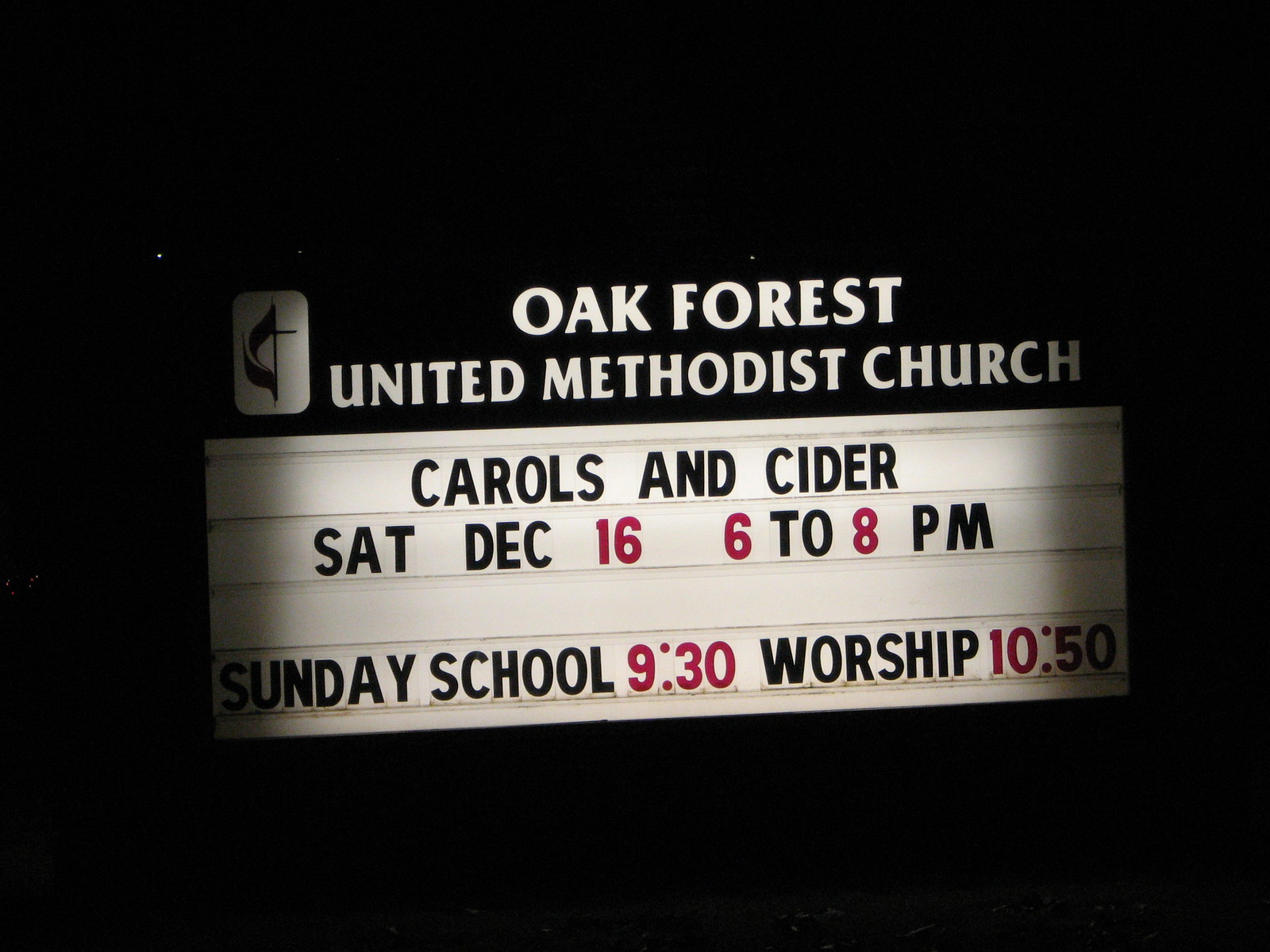This nighttime, color photograph captures the illuminated sign of Oak Forest United Methodist Church, positioned centrally in a landscape orientation. The rectangular sign glows with internal backlighting, standing out sharply against the surrounding darkness. The top portion of the sign features a black banner with white text that reads "Oak Forest United Methodist Church" and includes a white rectangle in the top left corner displaying a cross with a stylized red banner draped from top to bottom. Below this, the sign is a changeable letter board, where black and red letters spell out upcoming events and services: "Carols and Cider, Saturday, December 16th, 6-8 p.m.," followed by "Sunday School, 930 Worship, 1050." The sign has a black border around it, with its brightest illumination in the center, gradually dimming toward the edges, creating a fade into shadows. The realism of the photograph highlights the clear and practical design of the sign amidst the nocturnal setting.